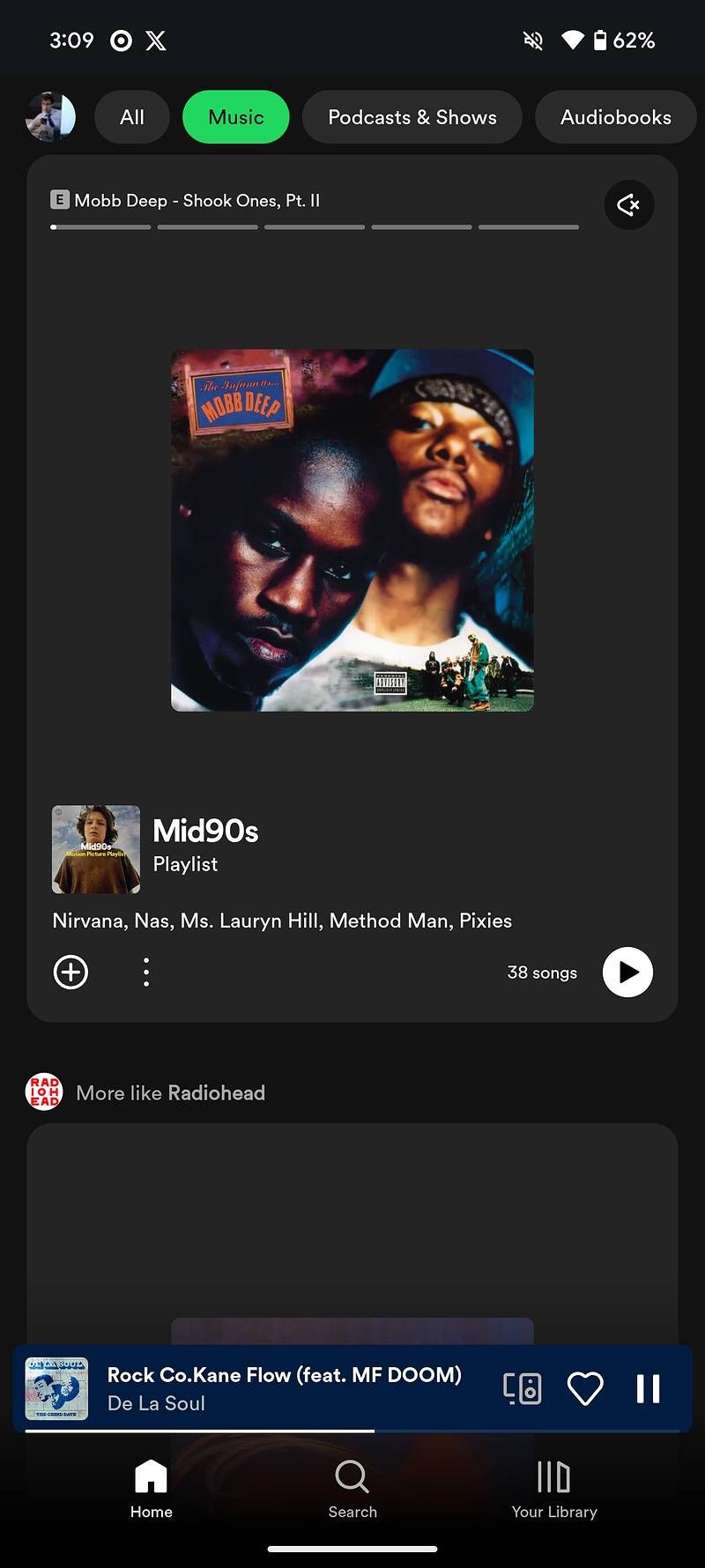The image is a screenshot of a mobile website, likely a music or audio streaming service such as Spotify. At the top of the screen, a menu bar is displayed with various buttons, all in black, labeled "All," "Music," "Podcasts & Shows," and "Audiobooks." The "Music" button is selected and highlighted in green. Below the menu, there is a section featuring an album cover that depicts a close-up of the faces of two young Black men standing side by side. Superimposed on the bottom left corner of this image is a scene showing a group of people gathered outdoors, possibly near a park bench. Below the album cover, there is a user-generated playlist titled "Mid-90s Playlist," which includes artists such as Nirvana, Miss Lauryn Hill, Method Man, and Pixies.